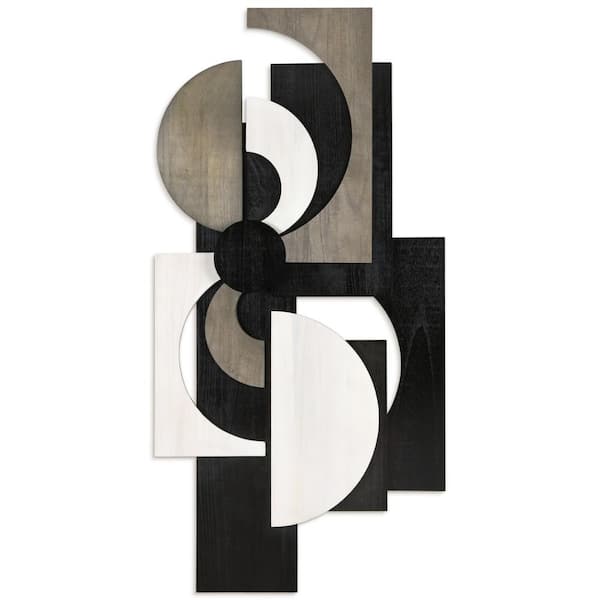The vertical image showcases a modern, multicolored wall art piece set against a plain white background, with a soft shadow suggesting it is mounted on a wall. This artwork, constructed from wood, features a variety of rectangular and circular shapes, including squares, circles, and half circles. The pieces display a range of colors from dark gray and muted brown to off-white or cream, and the wood grain texture is visible on some of the elements. At the bottom of the composition is a black rectangle, across which lies a white half circle and its negative counterpart—a black half circle cutout. Above this are two gray pieces: one with a half circle cutout and a smaller, separate half circle. Near the upper middle or middle left part of the artwork, a circular black shape integrates these components, enhancing its modern and simplistic design.